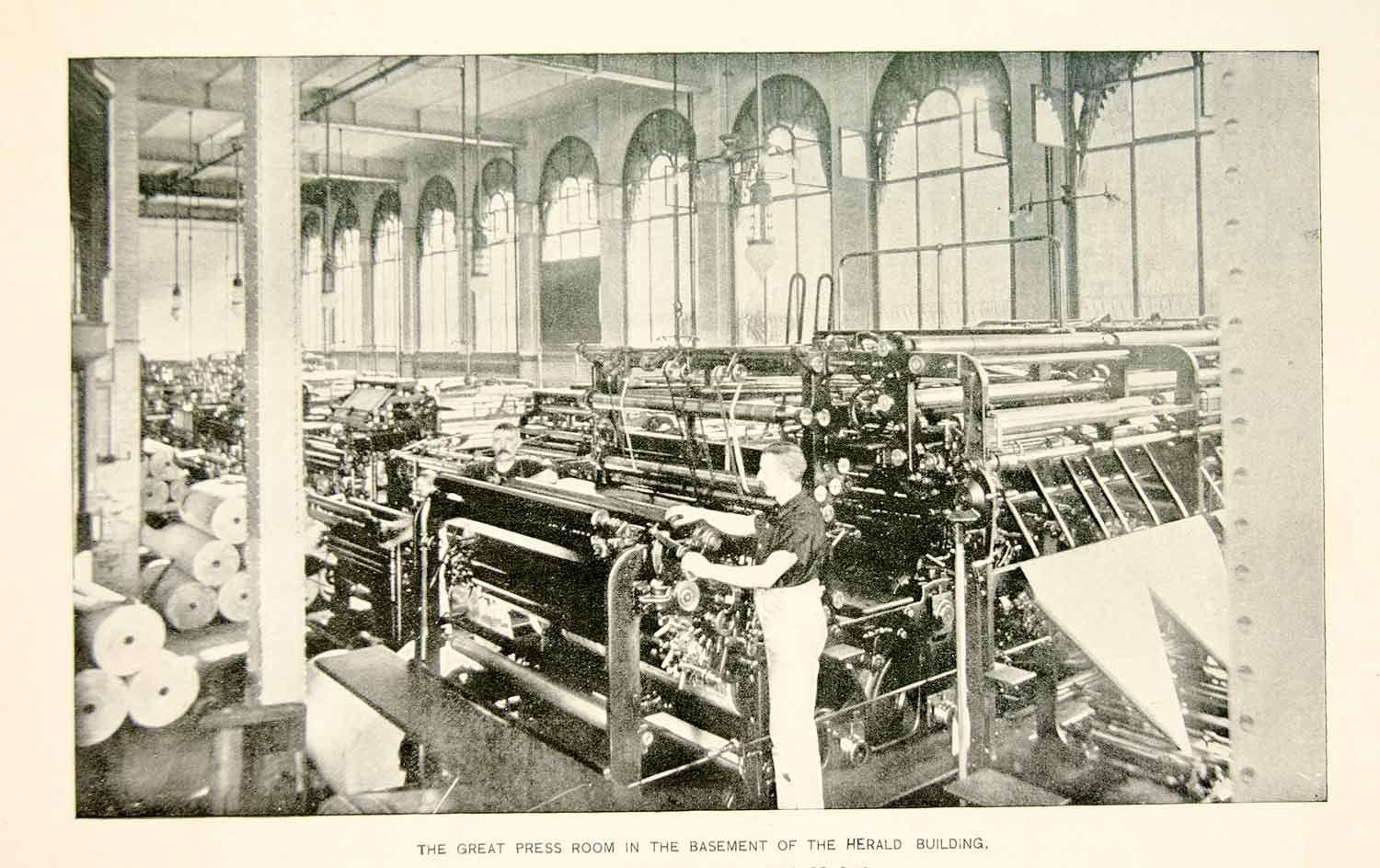This sepia-toned, black-and-white vintage photograph captures the bustling activity in "The Great Press Room in the Basement of the Herald Building," a historical newspaper manufacturing plant. The expansive room is filled with an array of intricate printing press machines, with stacks of paper rolls prominently displayed on the left side. The ceiling is adorned with light fixtures that hang down the center, illuminating the space. Tall, arched cathedral windows line the right wall, allowing a flood of natural light to accentuate the mechanical details of the presses.

Central to the scene is a clean-cut gentleman, meticulously working at one of the printing presses. He is dressed in high-waisted white pants and a short-sleeved, button-down, dark-colored shirt, with short hair, standing facing left. Another man, with dark hair and a mustache, can be seen working on a machine on the other side of the press. Both men, along with the meticulously arranged equipment and ambient industrial architecture, encapsulate the diligent atmosphere of this historic press room.